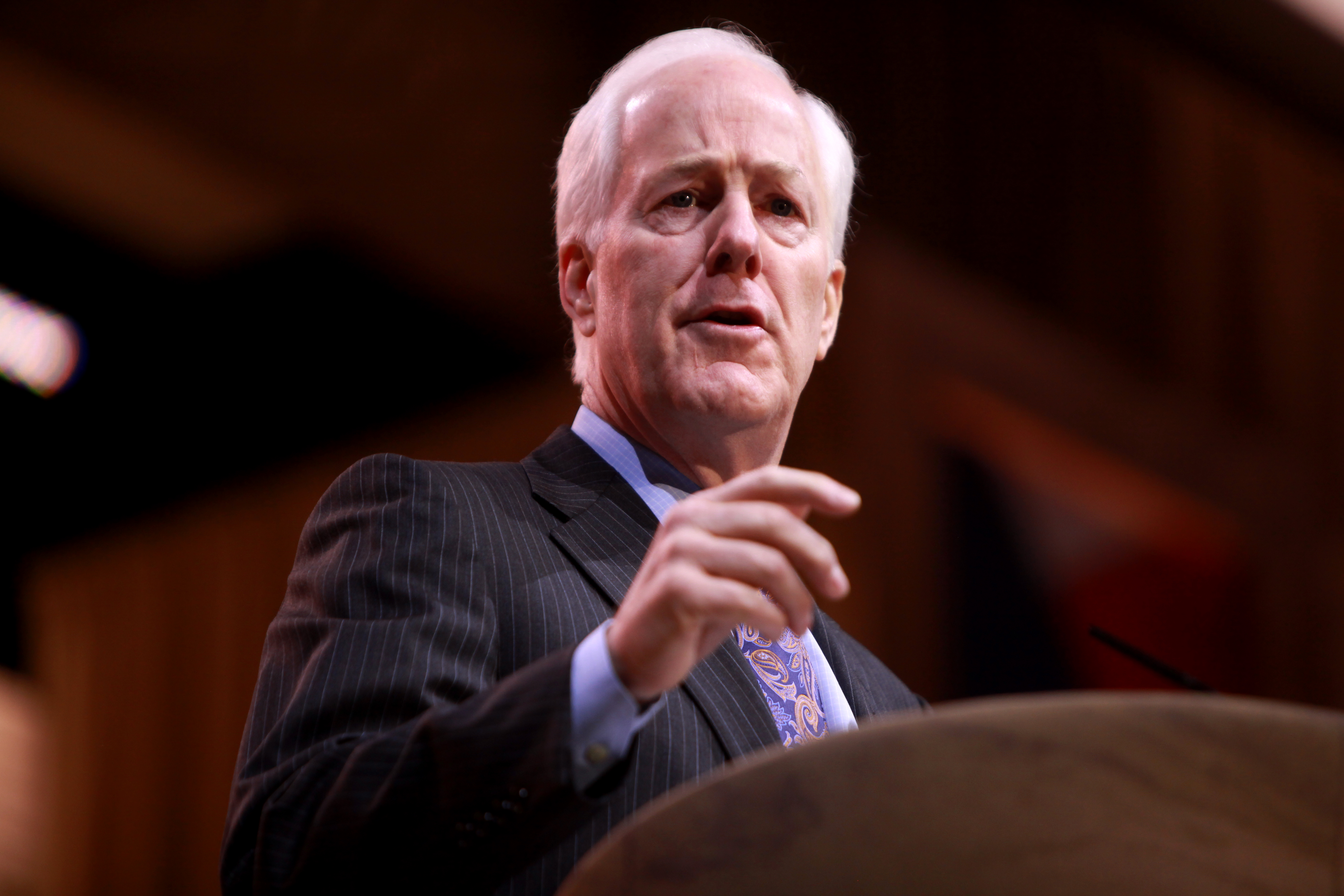The image presents an older white male, likely a politician or community leader, positioned centrally, speaking at a brown podium with a microphone. He appears to be in his 60s to early 70s. The man has white hair parted to the side, and he is dressed in a dark pinstriped suit with gray thin vertical lines. He wears a light blue shirt, with its collar and sleeves visible, and a patterned tie in shades of blue, purple, and possibly gold or orange designs. His right hand is raised as he gesticulates while speaking, his mouth open and his expression serious yet slightly confused. The background is dark, composed of brown and red hues, possibly indicating a wooden wall, but it is blurred out. The setting suggests a political conference or forum.